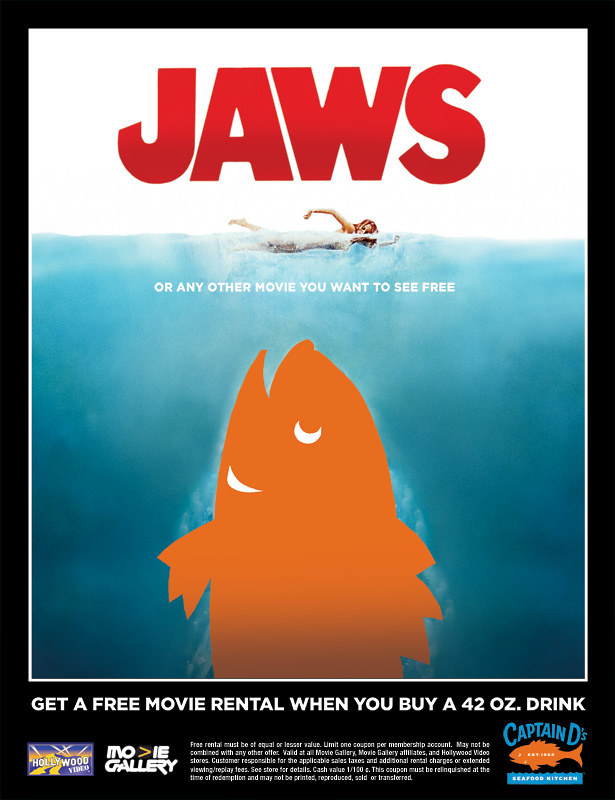This is a vintage magazine advertisement featuring a parody poster of the classic Jaws movie to promote a special offer. At the center of the ad, there's a humorous adaptation of the iconic Jaws poster: a woman with reddish hair swims across the white background from left to right, with the text "or any other movie you want to see free" situated directly below her. Instead of the menacing shark, a cartoonish orange fish from Captain D's logo, complete with white eyes and gill, mimics the shark's position, its mouth open wide as if approaching the swimmer.

The bottom section of the ad displays a striking black background with the bold text, "Get a free movie rental when you buy a 42 oz drink." To the bottom left, the logos of Hollywood Video and Movie Gallery are displayed side by side, while the Captain D's logo, featuring the same orange fish, appears on the bottom right. Additional small text below the logos outlines the promotion's terms and conditions, stating that the free rental must be of equal or lesser value and cannot be combined with any other offers. It also specifies that the coupon is valid at Movie Gallery, its affiliates, and Hollywood Video stores. The entire layout effectively merges the Jaws parody with a promotion deal by Captain D's, Movie Gallery, and Hollywood Video, making for a memorable and eye-catching advertisement.